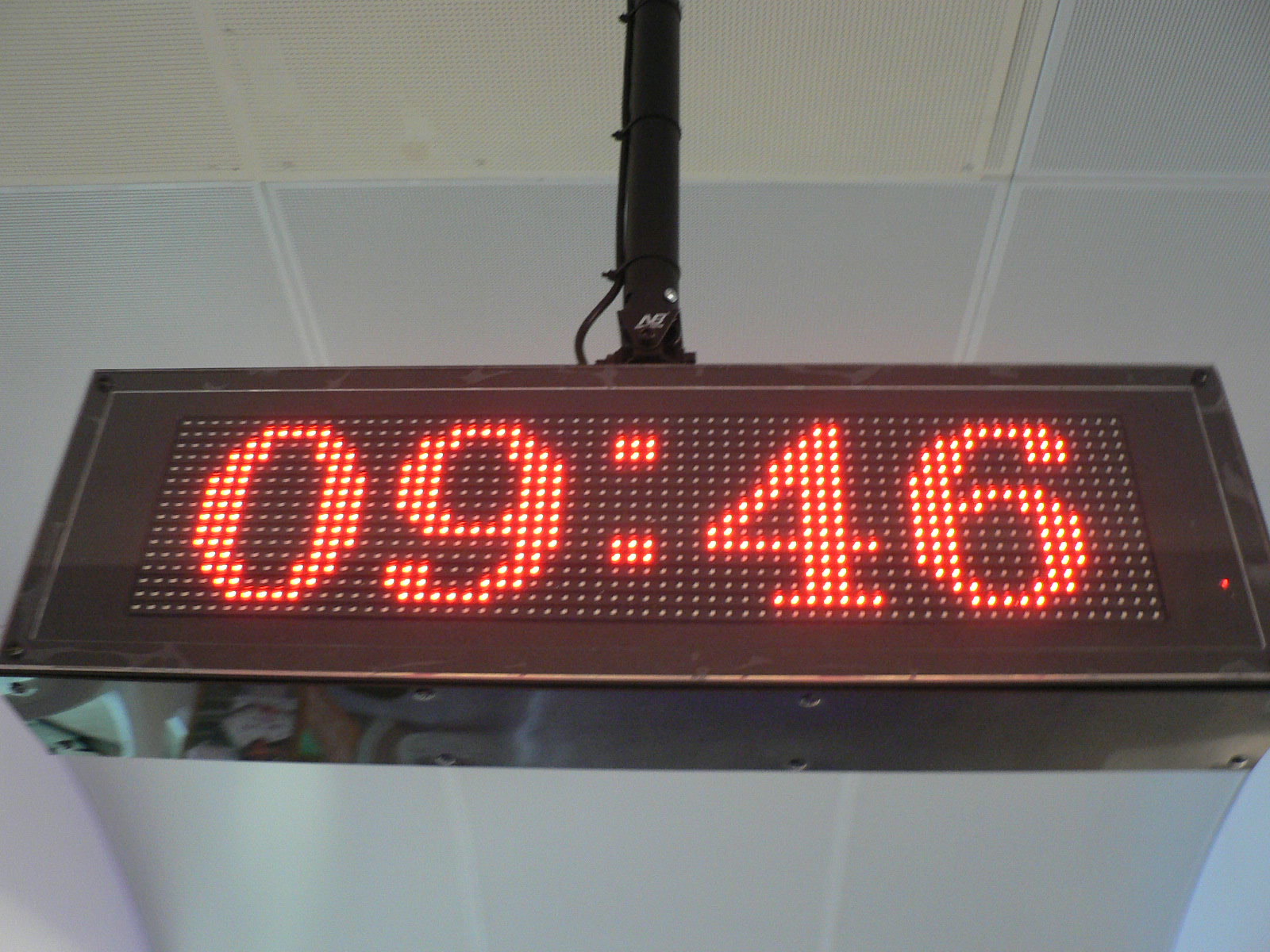This photograph captures a timing device suspended from a drop ceiling commonly found in office spaces or business buildings. The ceiling is composed of mostly white tiles, with a few tiles in an off-white hue. The clock is supported by a black mounting bracket attached to the ceiling.

The clock itself is predominantly made of a sleek, silver metal that resembles stainless steel. Its design is characterized by a long rectangular shape with a metal grate situated at the center, covering the digital display. The digital readout is backlit and features large numbers in a yellow color, outlined with red or orange, making it highly visible. The display currently shows the time as 09:46, with a semicolon separating the hours and minutes.